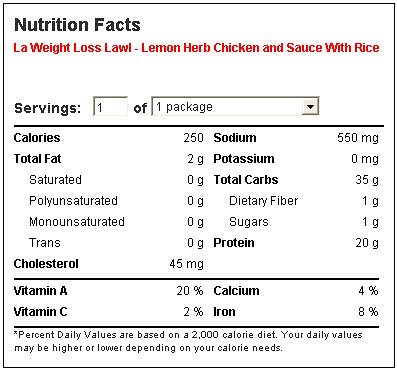This image depicts a digital representation of a Nutrition Facts label, resembling a late 90s or early 2000s computer interface. The label is primarily black and white, featuring "Nutrition Facts" prominently at the top in black text. Below that, highlighted in red, is the product name: "LA Weight Loss - LAWL - Lemon Herb Chicken and Sauce with Rice." The label includes an interactive section where the user can input the number of servings, currently set to one package. Detailed nutritional information is provided: 250 calories, 550 milligrams of sodium, 35 grams of total carbohydrates, 20 grams of protein, 45 milligrams of cholesterol, 0 grams of unsaturated fat, 5 grams of saturated fat, 0 grams of trans fat, 1 gram of sugars, 20% of the daily value for Vitamin A, 4% for calcium, 2% for Vitamin C, and 8% for iron. It's noted that the Percent Daily Values are based on a 2,000 calorie diet and that individual daily values may vary based on calorie needs.